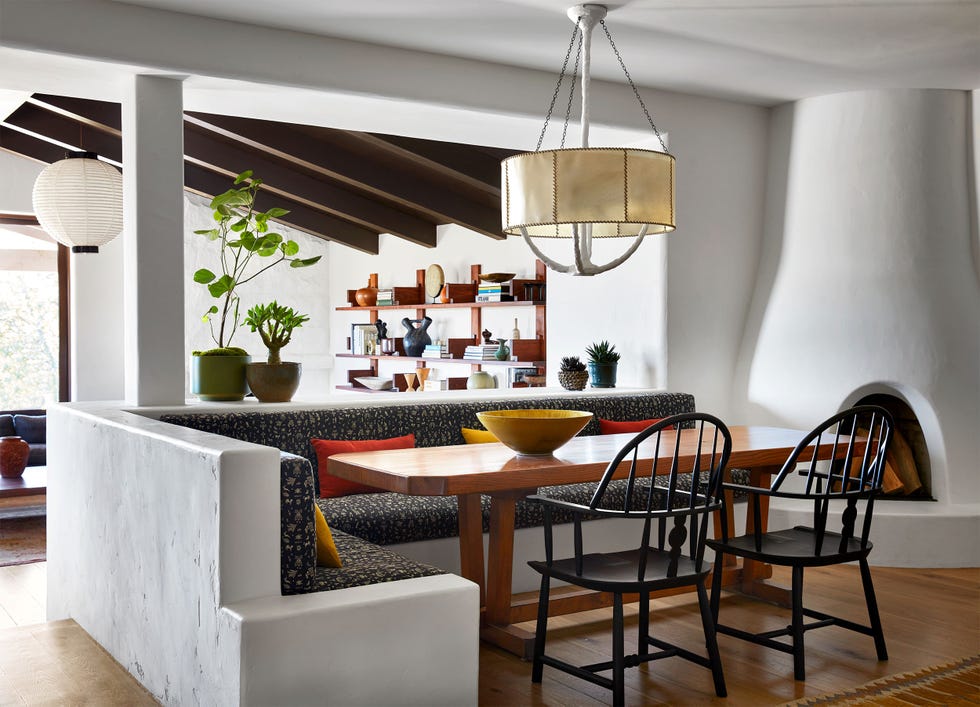This photograph showcases a beautifully detailed adobe-style dining room and adjacent living area within a house. The dining room features white plaster walls and an L-shaped built-in banquette upholstered with cushions that have a mix of brown, beige, and blue prints, complemented by mustard, yellow, and orange throw pillows. Central to this cozy nook is a rustic, light wood table flanked by dark wood ladder-back chairs. A large, mustard-yellow vase sits prominently on the table.

Adjacent to the dining area, a white built-in adobe-style fireplace with a small opening is seamlessly integrated into the wall. Above the table hangs a modern beige chandelier with a screen cover. The dining area transitions into a living space with dark wood rafter ceilings and wooden floors. In the background, potted plants and various knickknacks adorn a shelving unit, and a navy-blue sofa is faintly visible beside a large picture window. Rounding out the details, the room features additional lighting with round, balloon-shaped lampshades hanging from the rafters, adding a subtle touch of whimsy to the elegant yet cozy atmosphere.